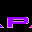The image is a very small icon-sized photo, less than half an inch square, featuring a black background. At the center, there is a prominently displayed purple letter "P", outlined subtly in yellowish-orange. The bottom left corner of the image shows a partial purple triangle, while the bottom right corner has a small segment of a red triangle. Despite zooming in, details remain limited, suggesting it could be a cropped screenshot of a larger text. The overall aesthetic of the photo seems reminiscent of a digital 80s style format.